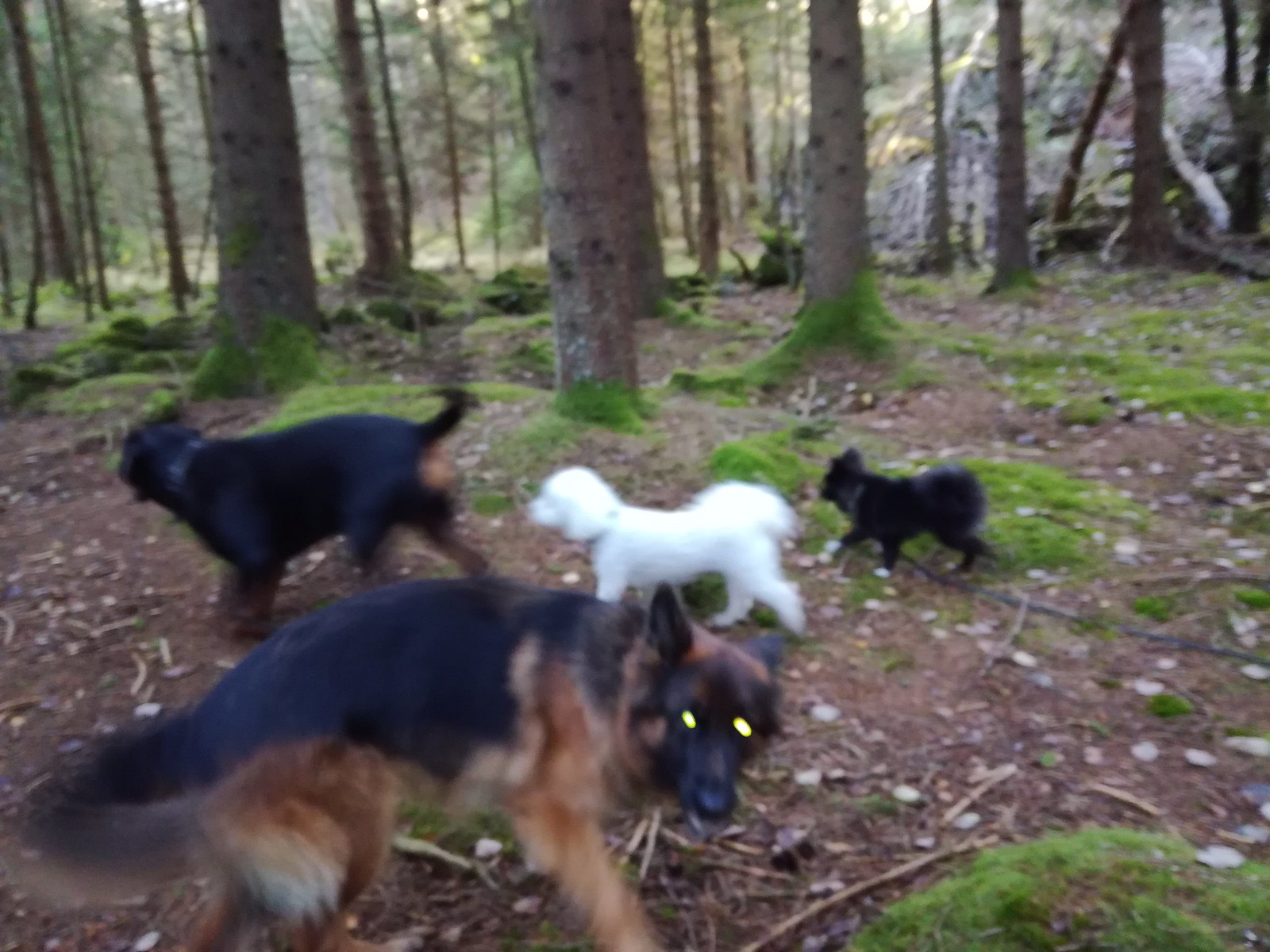This outdoor photograph, taken during the daytime in a wooded area, captures a slightly blurry scene with four distinct dogs. The background features the lower trunks of numerous trees and a brush pile of several tree limbs in the upper right-hand corner. The ground is predominantly dirt with twigs, interspersed with patches of moss and small rocky outcroppings.

Dominating the foreground is a German Shepherd with a black and brown coat, gazing directly at the camera with striking, glowing yellow eyes. Trailing behind him to the left are three other dogs: a large black dog with brown spots, which could be a Rottweiler; a medium-sized fluffy white poodle wearing a collar; and a small black dog, possibly a Pomeranian. The latter three dogs are all heading towards the left of the image, appearing to move away from the camera. The slight blurriness and out-of-focus elements suggest the photo was taken in a low-light setting with considerable movement, enhancing the natural, lively atmosphere of the scene.